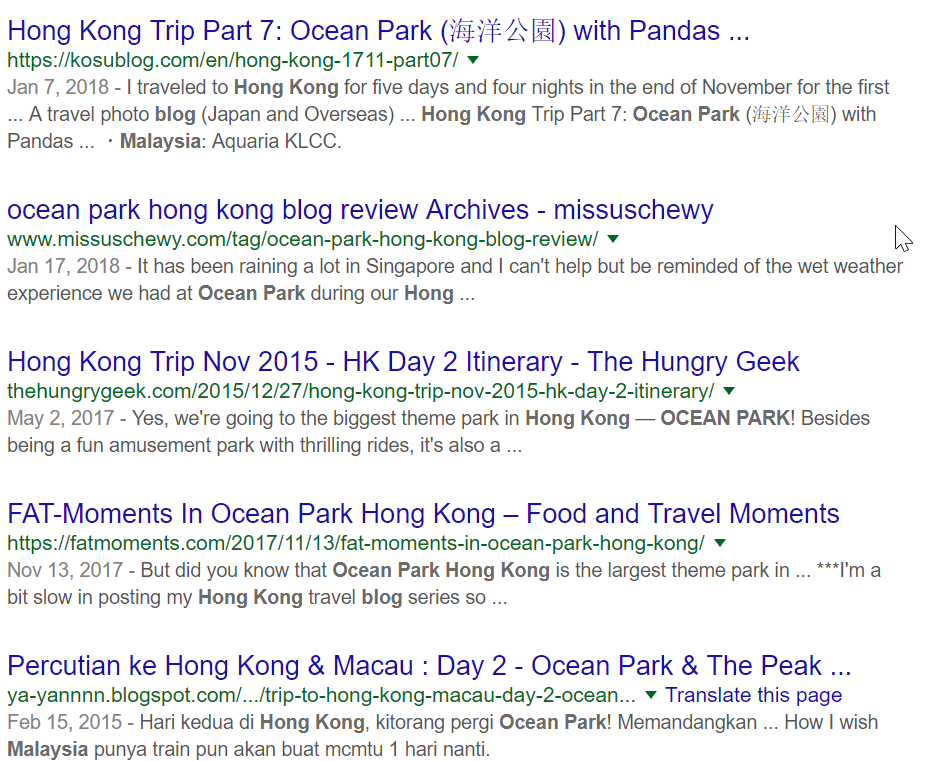The image showcases a resource reference webpage dedicated to a Hong Kong trip, prominently featuring blog posts and articles related to Ocean Park. The first highlighted section, titled "Hong Kong Trip Part 7: Ocean Park," includes Asian script and images of pandas. The description mentions a travel date of January 7, 2018, and notes, "I traveled to Hong Kong for five days and four nights in late November," though the text cuts off, prompting users to click for more details. This section belongs to the "Ocean Park Hong Kong Blog Review Archives" by Missus Chewy, dated January 17, 2018.

Following this, there are several other sections:
- "Hong Kong Trip 2015 HK Day 2 Itinerary" by The Hungry Geek.
- "A Fat Moment in Ocean Park Hong Kong: Food and Travel Moments."
- "Percussion Key: Hong Kong and Macau, Day 2: Ocean Park and the Peak."

Each of these sections is written in a purplish color and includes short descriptions beneath, detailing the contents of the respective articles. The webpage lacks a search bar, and the method of how this information was compiled is unclear, but all listed items are clickable for further reading.